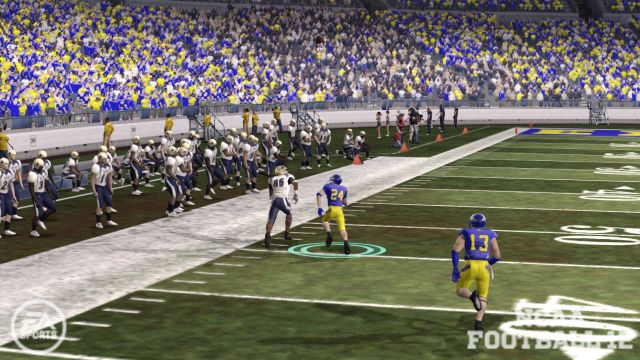The image is a detailed screenshot from the video game "NCAA Football 12," capturing a tense moment on a dark green football field. In the foreground, we see two players in purple jerseys with yellow numbers and yellow pants, alongside a player in a white jersey with black pants, likely holding the ball. The players are positioned around the 40-yard line, with one player in white near the sideline. The background reveals a photorealistic representation of a crowded stadium, filled mostly with fans in purple and yellow, signifying strong support for one of the teams. The bottom corners of the screen feature the game's title, "NCAA Football 12," and the EA Sports logo in gray, transparent text, reinforcing the game's branding. The combined vibrancy of the player's uniforms and the animated crowd captures the dynamic atmosphere of a real-life football game, despite being a virtual depiction.